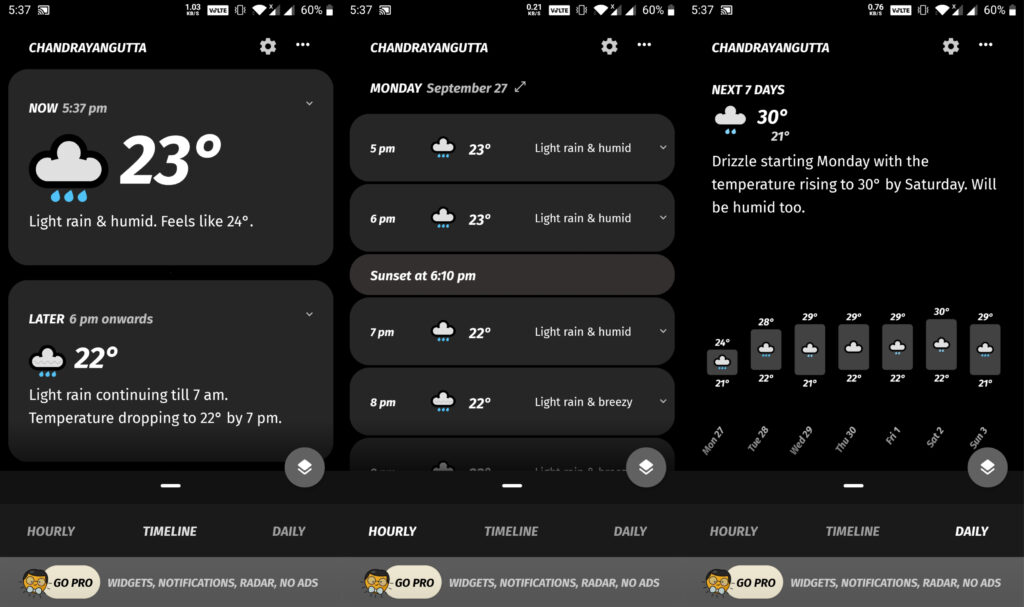Here is a detailed and cleaned-up caption for the described image:

---

This image showcases a collection of three mobile screenshots from a weather app, displayed side by side in a horizontal row. Each screenshot features a consistent black background, indicative of night mode on the phone. The top left corner of all three screenshots shows the time as 5:37 PM, while the status bar on the top right corner displays the same icons and battery percentage across all screenshots.

The first screenshot on the left highlights the weather for the area called Shandrayangatta. A cogwheel icon and a menu box are positioned to the right of the area name. Below this, a lighter-colored black box states "Now, 5:37 PM." Beneath this, a rain cloud icon with raindrops is displayed next to a large white text reading "23°." Further down, the text "Light rain and humid, feels like 24°" is provided. In addition, a box labeled "Later, 6 PM onwards" describes the weather forecast as light rain continuing until 7 AM, with the temperature dropping to 22° by 7 PM.

The middle screenshot offers a vertical listing of the day's weather for Monday, September 27th. It starts with "5:00 PM, 23°, Light rain and humid," followed by "6:00 PM, Sunset at 6:10 PM," and continues with details for "7:00 PM" and "8:00 PM."

The third screenshot on the far right presents the weather forecast for the next seven days. It mentions a high of 30° and a low of 21°, indicating rainy conditions with drizzles starting Monday. The temperature is predicted to increase to 30° by Saturday, which is also expected to be humid. At the bottom, a horizontal list illustrates the highs and lows for the week, with specific dates provided underneath.

---

This caption provides a clear and detailed description of the content within each of the three screenshots.